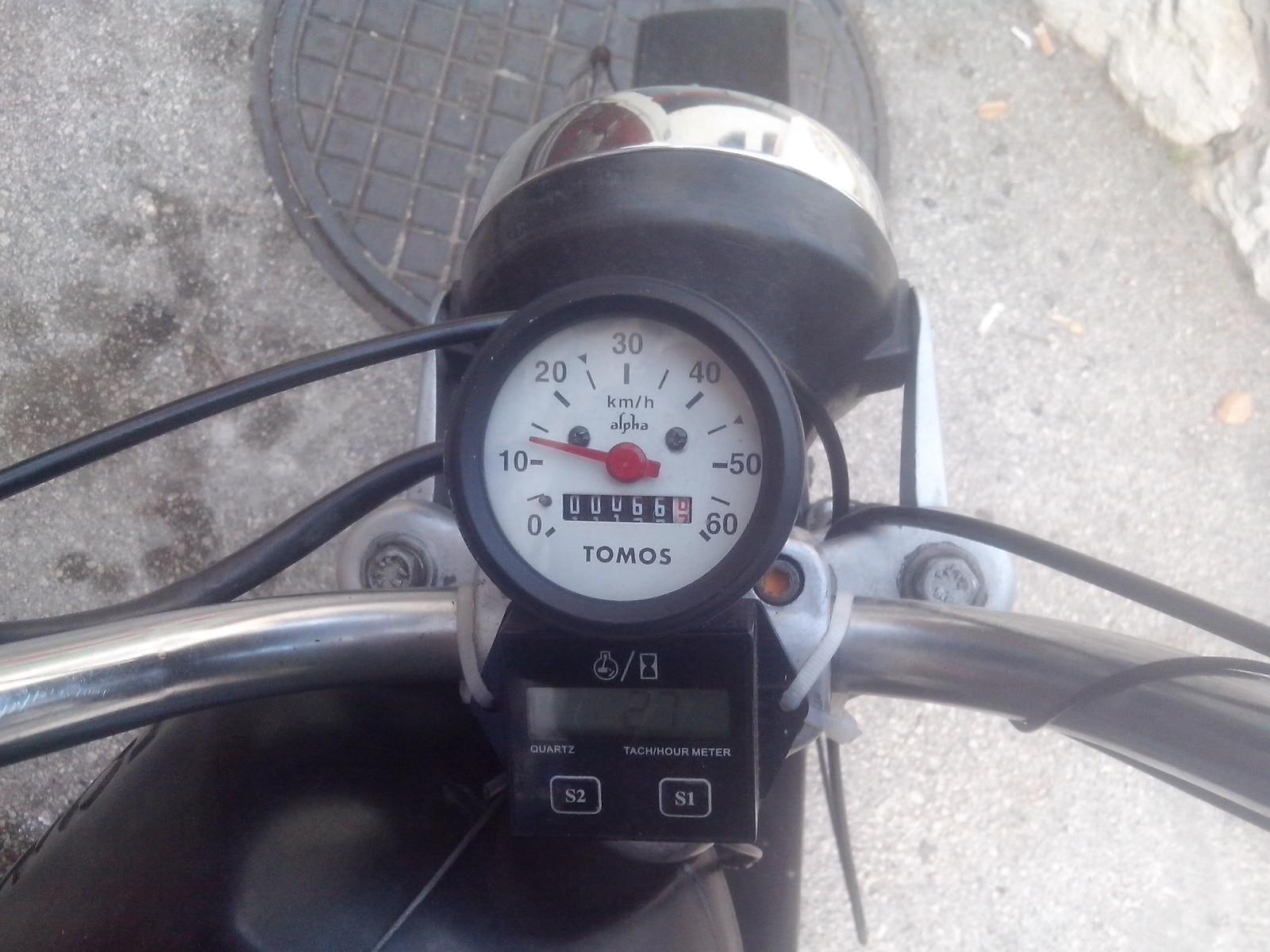A motorcycle is positioned prominently on the road, showcasing its front features and the surrounding environment in vivid detail. The main focal point is its large black front tire, accompanied by a close-up view of the silver components near the tire. Above this, a detailed speedometer with a white face and black numbers indicates speed in kilometers per hour, also displaying 66 miles on a small rolling counter. The speedometer bears the inscription "TOMAS" in black letters at its base. Adjacent to the speedometer, there is a black panel featuring several white symbols, alongside a quartz tachometer meter marked with "S2" and "S1" within black squares bordered in silver. The motorcycle's handlebars are visible, with wires neatly wrapped around them.

The road in the background reveals a patchwork of pavement, marred by an abundance of oil stains and dotted with cigarette butts on the right side. A prominent manhole cover for the water mains sits at the center, surrounded by scattered white rocks near the roadside. This image conveys the rugged, detailed context of a typical street scene, contrasted with the precise and intricate design of the motorcycle's front section.